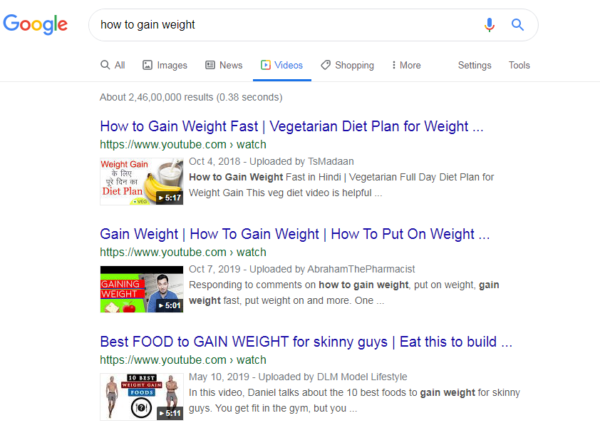The image is a screenshot of a Google search page. In the upper left corner, the Google logo is prominently displayed, and to its right, a search field is visible with the query "how to gain weight" entered. To the far right of the search field, there is a microphone icon, which users can click to verbalize their search instead of typing, followed by a small magnifying glass icon indicating the search function.

Below the search field, there are several menu options. From left to right, these options include: "All," "Images," "News," "Videos" (which is currently selected), "Shopping," "More," "Settings," and "Tools." The selected "Videos" option is highlighted in blue with a blue underline, while the other options are in black font.

Further down, you can see the typical layout of Google search results. The page indicates that there are approximately 2.46 million results for the search query, displayed in small, grey font. The first result appears in blue font, titled "How to Gain Weight Fast: Vegetarian Diet Plan." The second result is similarly formatted and titled "Gain Weight: How to Gain Weight, How to Put On Weight." The third result reads "Best Food to Gain Weight for Skinny Guys."